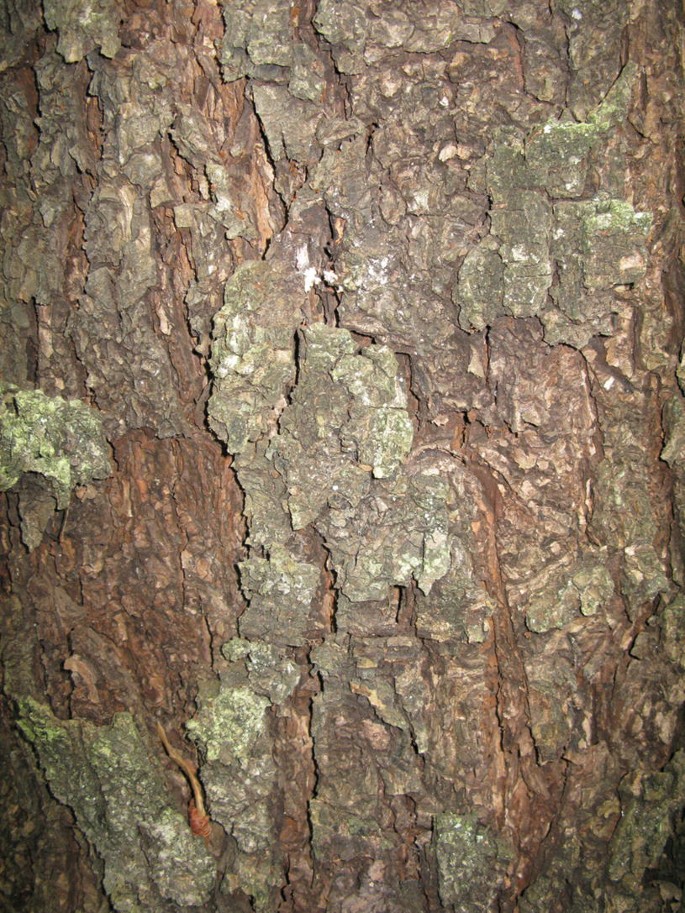The image is a close-up, portrait-orientation color photograph completely filled with the rugged, chunky bark of a pine tree. The bark displays varying shades of light brown, with patches of exfoliated areas revealing the smoother, deeper brown wood underneath. There are growths of green and white lichen scattered across the surface, adding texture and color contrast. In certain areas, the lichen-covered bark has sloughed off, providing glimpses of the smoother, non-lichenized bark below. The overall appearance is quite detailed and textured, with visible layers and peeling sections of bark. Additionally, towards the bottom left corner of the photograph, there appears to be a small orange worm or similar creature nestled between the pieces of bark, further contributing to the intricate and natural complexity of the image.